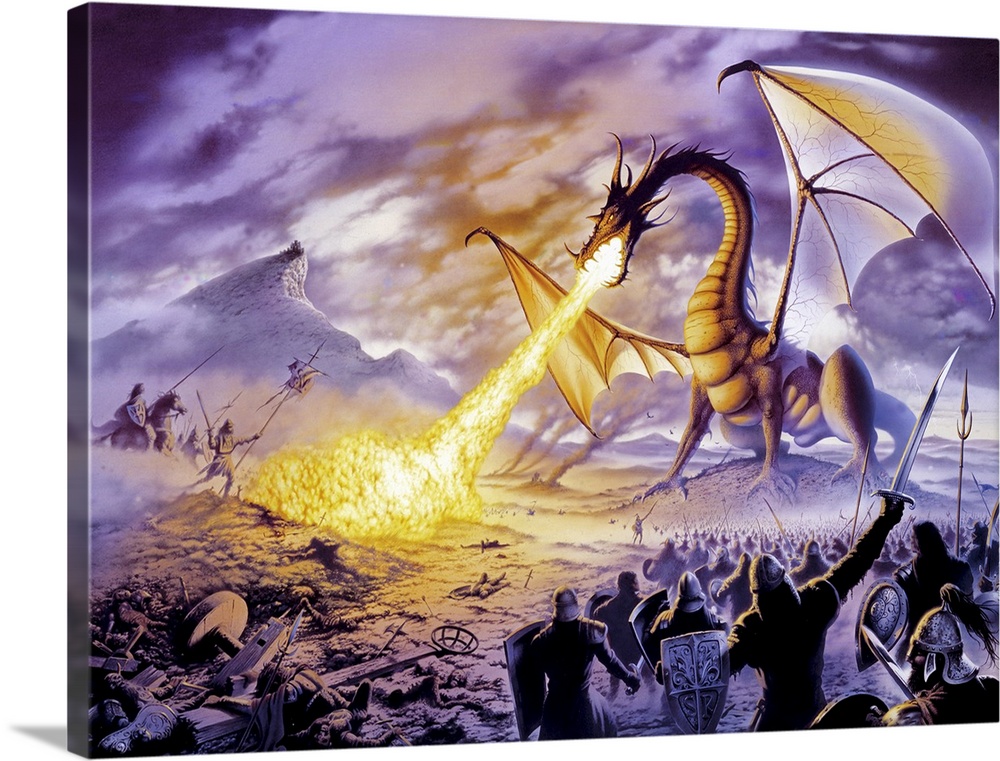In this detailed color illustration, displayed in landscape orientation, a dynamic and fiery battle scene unfolds between humans and a formidable dragon. The canvas, slightly tilted to reveal its left edge, captures the viewer's attention immediately. 

Dominating the upper right quadrant of the image, the yellowish dragon, with its translucent, whitish wings outstretched, releases a blazing stream of fire from its mouth. The dragon's curved neck and fierce expression add to its menacing presence as it perches on a slight, snow-covered mound in the foreground. The fiery stream arcs towards the lower left center, creating a dramatic focal point.

Below, on the right side of the scene, a mass of soldiers stands in defiance. They wear hard silver helmets and armor, holding their shields up and swords raised above their heads. Closer to the center-left, another group of armed men and a few mounted on horses brace themselves for the onslaught. A particularly brave individual charges ahead with a standard flag, leading the defense.

The background is painted in varied hues of dark purple, black, and orange, depicting a tumultuous sky and the glow of the dragon's fire. A towering mountain peak with a discernible structure atop it rises on the left side, contributing a sense of scale and depth to the scene. The snowy landscape on the bottom left adds a cold contrast to the fiery chaos, where a catapult-like device aims towards the dragon.

This fantasy-themed illustration, rich in color and detail, vividly portrays the epic confrontation amid a purplish twilight setting.